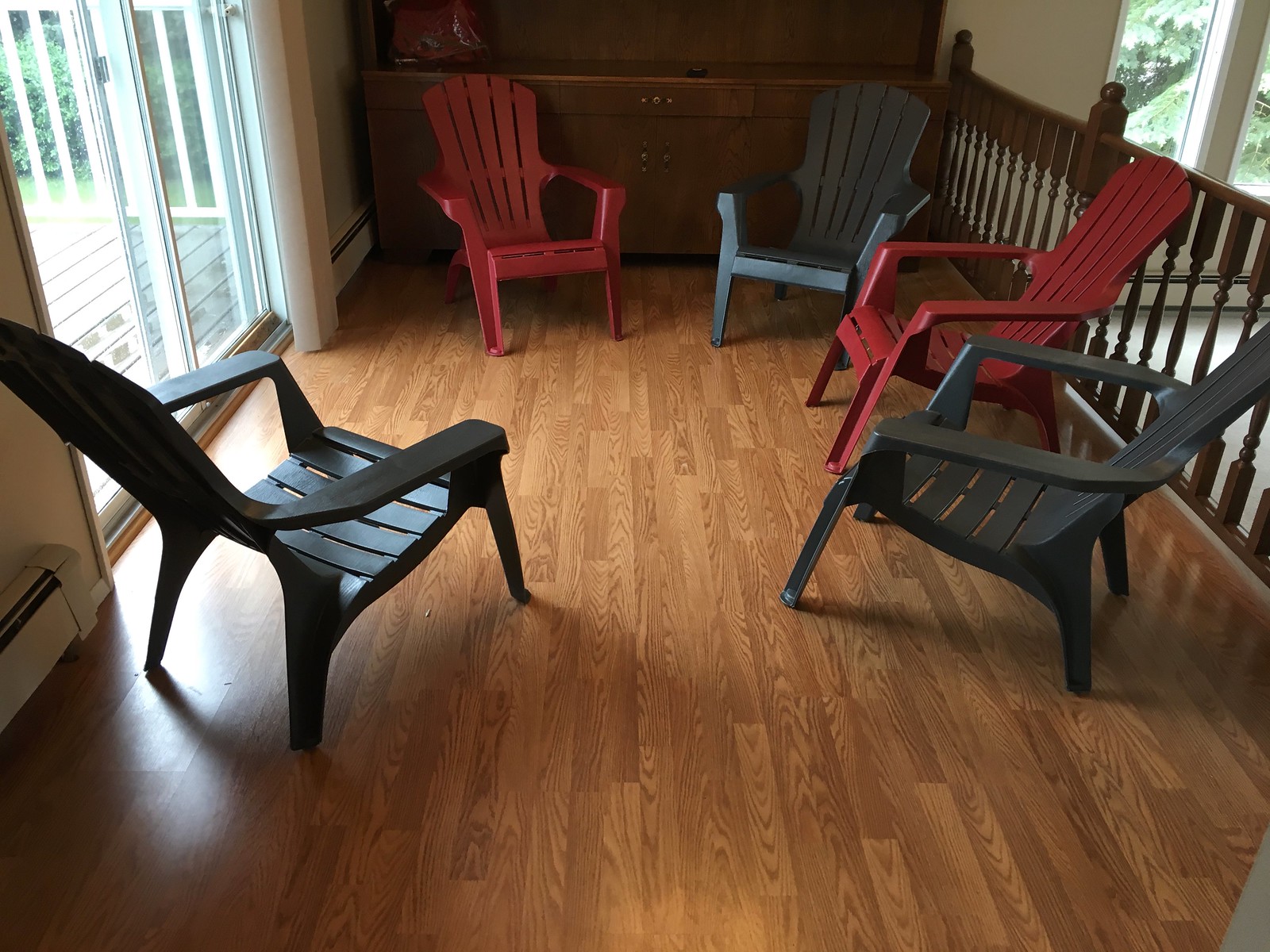This image captures a small, sparsely decorated interior room with notable features and furniture arrangement. The room has a dark brown hardwood or parquet floor and a dark brown wooden cabinet or hutch positioned against the back wall. On the right side, there is a decorative wooden railing, possibly leading to another room or indicating a stairway, with a beige wall behind it sporting white-framed windows flanked by a white baseboard heater beneath them. To the left, a white-framed sliding glass door offers a view outside, suggesting daytime lighting filtered into the room. Below this door is another white baseboard heater. Central to the image are five plastic Adirondack or Muskoka chairs arranged in a rough semicircle. Three chairs are dark gray, while the remaining two, placed on either end, are a dark brick red. These chairs provide the primary focal point in this clean and minimally furnished space.